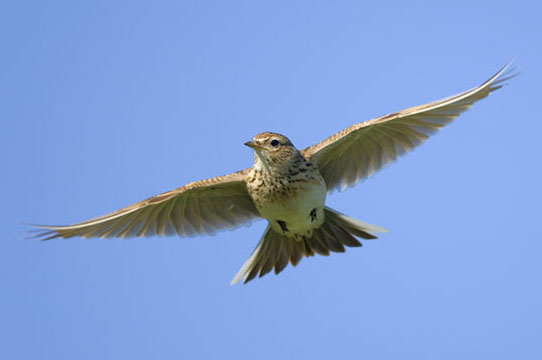In this detailed photograph, a medium-sized bird, roughly the size of a pigeon, is captured in mid-flight against a pristine, bright blue sky devoid of any clouds. The bird, facing slightly to the left, has both wings fully spread—its left wing extending towards the upper right corner and its right wing towards the lower left corner of the image. The bird is a mix of white and brown, with darker brown line segments adorning its chest, legs, and the sides of its wings. The bird's beak is tan, and its eyes are black. The head and upper body are predominantly brown, while the belly is light brown. Its short legs, which are tucked back, appear black. The bird's wide, short tail is also fully spread, showcasing its brown color. This solitary bird in the expansive, uncluttered sky brings forth a sense of freedom and tranquility.